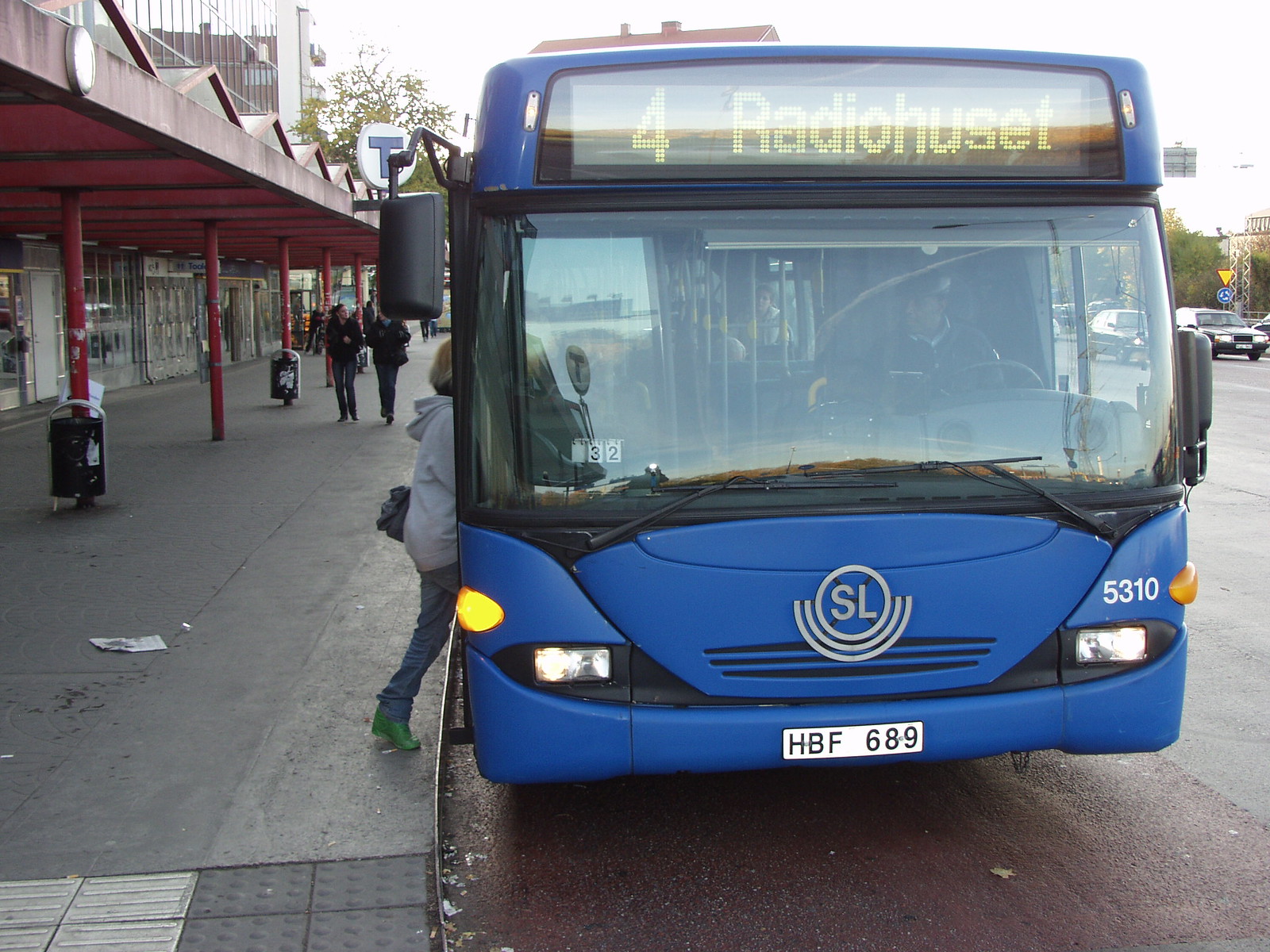The image depicts a bustling city scene at a bus stop. Dominating the foreground is a blue city bus marked with the number 4 and a display reading "Radio H-U-S-E-T." The bus's front is detailed with a large glass windshield, a circular emblem featuring the letters "SL" flanked by two half-circles, a stripe of blue around the bumper and headlights, and a license plate reading "HBF-689." A woman, clad in a gray hoodie, jeans, and green shoes, is seen boarding the bus. Behind her, the shelter of the bus stop is supported by several poles and features a protective roof. To the side, a busy sidewalk stretches ahead with pedestrians walking against the backdrop of storefronts adorned with a red awning. Some vehicles can also be seen passing by the bus on the adjacent roadway, suggesting a lively urban environment. The setting hints at an international location, suggested by the unfamiliar language on the bus display and license plate.